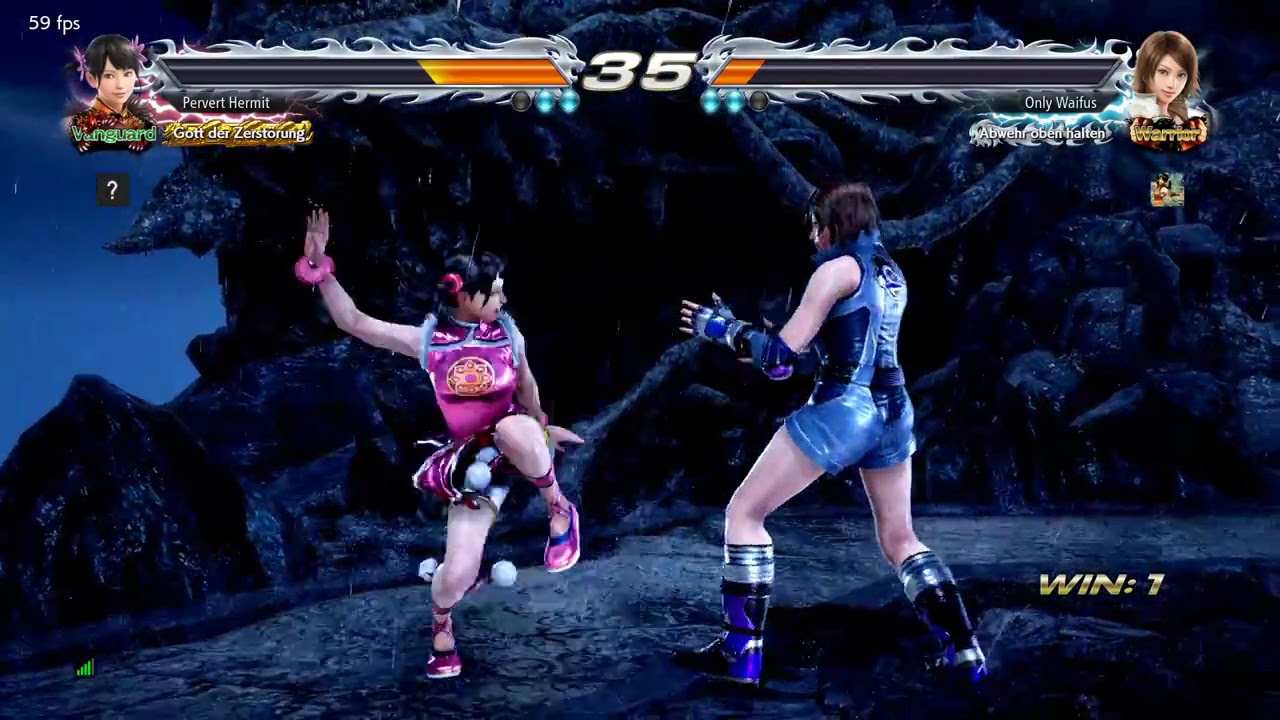The image is a detailed still photo of a fighting game, showcasing an intense battle between two feminine characters in the center foreground, framed by a dark blue and black background that hints at a mountainous or cavern-like setting. The left character, a woman with black hair adorned with a red flower, is dressed in a striking pink native outfit. Her right arm, decorated with a bright pink fuzzy bracelet, is raised above shoulder height, while her left arm is extended behind her. Positioned in a dynamic stance, her left leg is bent at the knee, seemingly prepared to kick her opponent, as her right leg remains stable. She is wearing sandals.

Her opponent to the right, whose gender is ambiguous as they are seen from the back, has black hair and is equipped in a blue combat outfit featuring a tank top, shorts, blue and black gauntlet-type gloves, and boots trimmed with silver edging. This character lunges forward on their left leg, their left arm bent and extending toward the opponent.

Above the fighters, a black horizontal bar with white flames in the top center of the image displays the number 35, likely indicating the score or time. Flanking the bar are avatars of the combatants, clearly marking their positions. In the lower right corner, a black rectangle with gold writing reads "Win: 7."

The image is vibrant with a palette that includes shades of blue, pink, black, gray, yellow, gold, orange, green, beige, light blue, and purple, emphasizing the game's digital artistry. Text within the image includes "59 FPS 35," "Vanguard," "Pervert," "Hermit," "Got der Zerstörung," "Only waifus," and "Win 7," further enriching the setting of this dynamic video game battle scene.